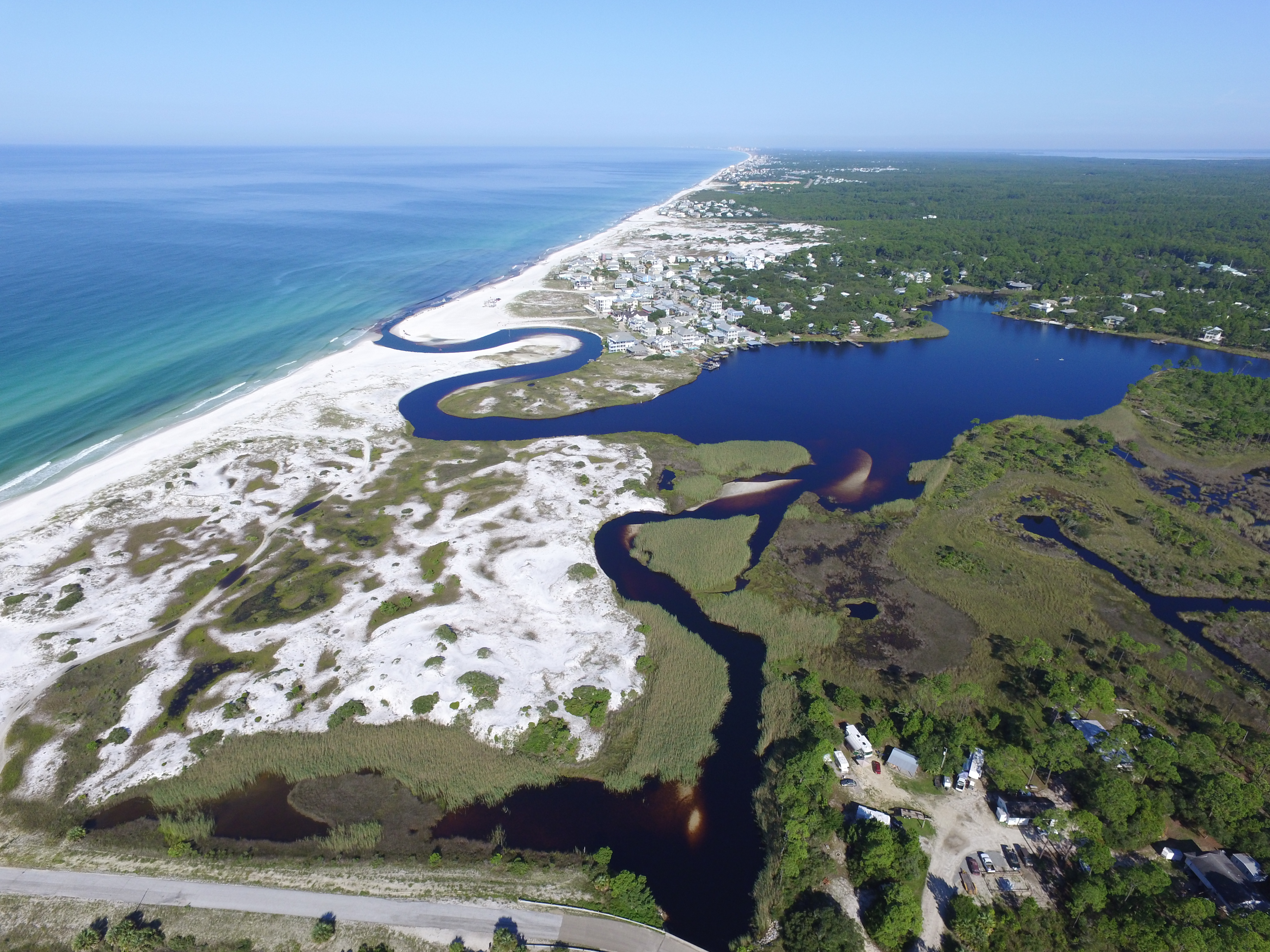This color aerial photograph captures a coastal beach town in remarkable detail, showcasing a vibrant landscape in a landscape orientation. To the top left of the image, the aqua-colored ocean extends diagonally towards the top right, bordered by a pristine white sandy beach closer to the center. Numerous trees dot the landscape, providing a lush backdrop to the scene. In the middle of the image lies a pond or retention area with dark blue water, shaped irregularly and connected to the ocean by an S-shaped canal. Another brackish water canal emanates from the retention area, branching towards the bottom center and then to the left. A gray paved road is visible on the bottom left, while patches of white sand are dispersed throughout the area. On the top part of the image, residential houses are nestled among the greenery, under a clear blue sky. Additionally, there is a parking lot situated on the bottom right side, with cars visible but no detectable presence of people or animals. This photograph epitomizes realism through its detailed depiction of the coastal landscape.